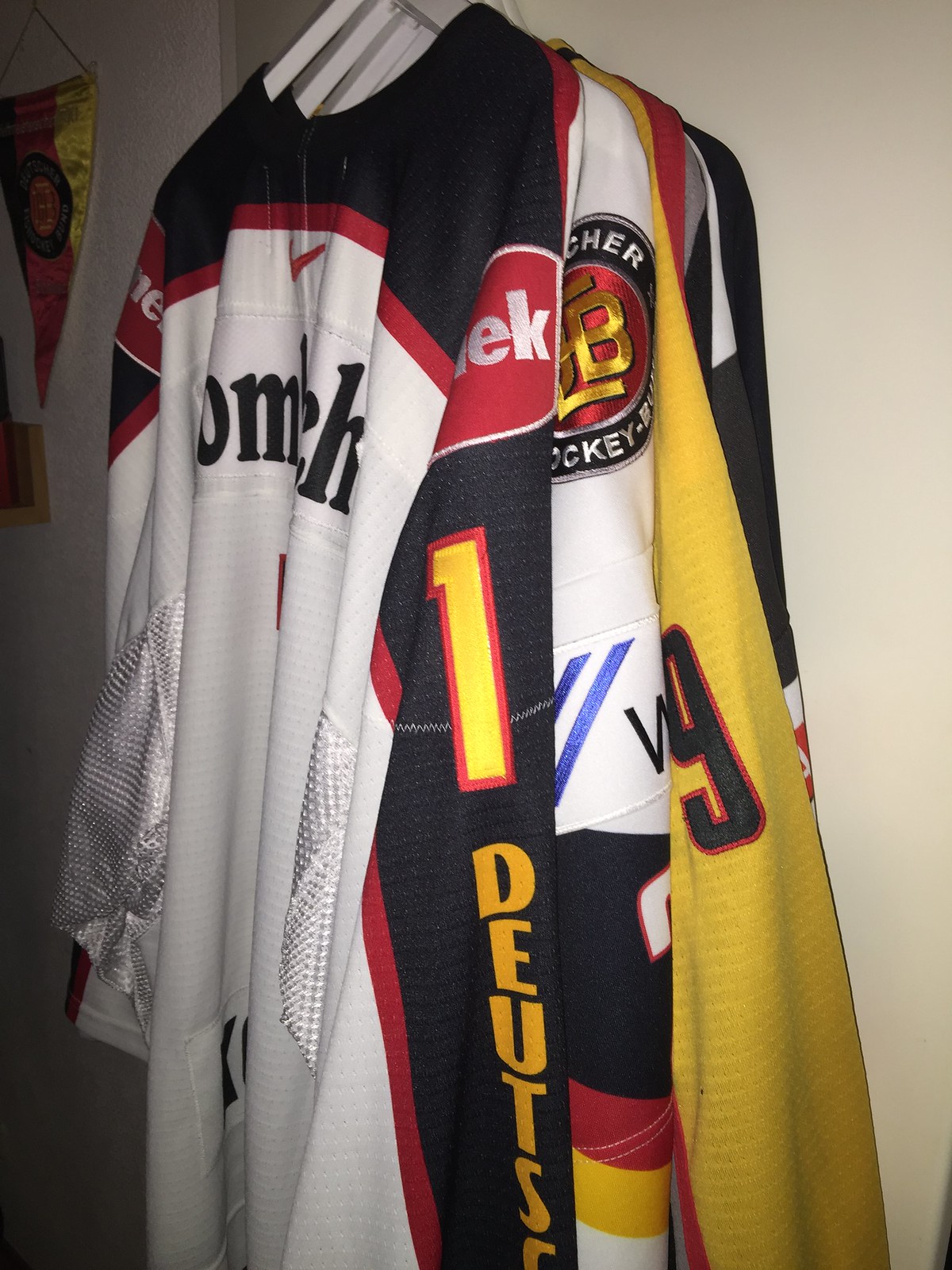In this image, we see a collection of German hockey jerseys hanging on a cream-colored door, with an off-white, rough-textured wall in the background. The jerseys appear vibrant and varied, suggesting team or player affiliations. Dominating the foreground is a predominantly white jersey with black sleeves and a bold yellow number "1" outlined in red on the sleeve, accompanied by the word "Deutsch" partially visible. Behind it, another jersey displays a German flag motif with diagonal blue stripes and a circular emblem featuring a black outer ring and a red inner circle with indistinct gold text. Additional jerseys, including a yellow one with a black number "9" outlined in red, and others with gray, black, and red accents, are also visible but partially obscured. Above, a pendant showcasing the German flag colors—black, red, and yellow—adorns the left side. The setting, featuring casual flag decor, suggests this might be someone's bedroom rather than a clothing store.